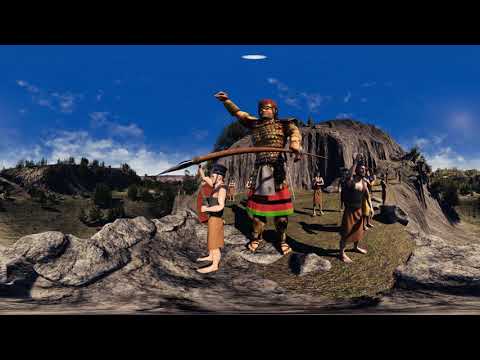This image, likely a screenshot from a video game or an art piece, depicts several historical or prehistorical figures standing on a rocky, grassy hill or mountain. The central figure is a towering, armored man holding a sword or spear, flanked by smaller individuals in old-fashioned, possibly Roman, attire with some raising their fists. The scene, set outdoors during the daytime, features a predominantly dark blue sky dotted with a few white clouds. Green tree-covered hills are visible on both sides in the background, and more people are lined up along the sides of the mountain. The mountains themselves are gray with yellowish grass, and the overall setting suggests a significant, historic moment captured on this elevated terrain. There is no text within the image, allowing the viewer to focus on the vibrant colors and detailed composition of the scene.